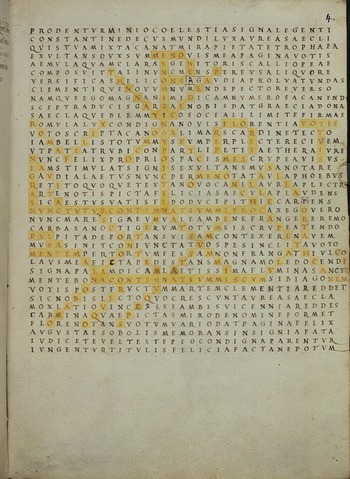The image features a word search puzzle, not a crossword, seemingly taken from a newspaper or magazine. The puzzle itself appears black and white, but overlaid on it is an intricate, modern design drawn with a yellow highlighter, suggesting someone turned the puzzle into a piece of art out of boredom. The highlighted design includes a ship-like figure with a large mast resembling a Norse symbol or rune, along with visible oars. Additionally, the design incorporates numerous X's and straight lines, creating a complex pattern. Select letters such as V-O-T or V-P-O-T might be visible, but it's unclear whether these connect to any discernible words or simply contribute to the artistic pattern.